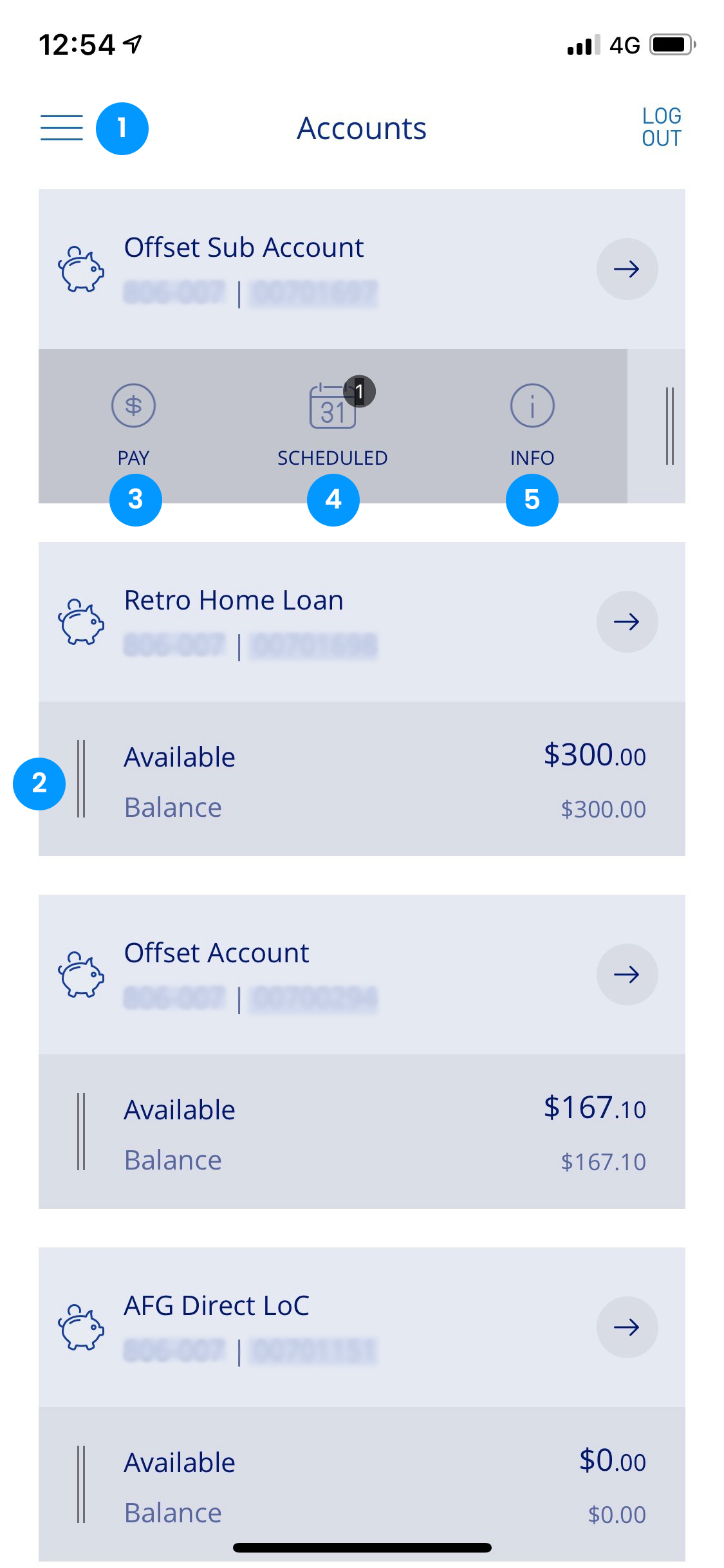The image is a screenshot of a cell phone screen, displaying a financial account management app. In the top left corner, the time reads 12:54. The top right corner shows a cellular data symbol, '4G' connectivity, and a mostly full battery icon. 

Below this status bar, there is a blue circle with the number '1' inside, next to the word "Accounts" followed by "Logout". The next section features a gray background with the text "Offset Sub Account" and an image that appears to be a logo of a pig, accompanied by an arrow pointing to the right.

Underneath, there is a circle with a dollar sign, labeled "Pay". To the right of this is a calendar icon with the number '31' and a '1' overlay. Below this reads "Scheduled". Further to the right is another circle containing the letter 'i', labeled "Info". 

Three circles span the screen, each containing a number: '3' in the first circle, '4' in the second, and '5' in the third. Below this sequence, the text "Retro Home Loan" is displayed, alongside the pig logo and another arrow pointing right.

Next, a blue circle with the number '2' is followed by the text "Available Balance $300". Another entry, labeled "Offset Account", follows, showing the pig logo and an arrow pointing right with an available balance of $167.10. Finally, the text "AFG Direct LOC" appears, paired with the pig logo and an arrow pointing right, indicating an available balance of $0.00.